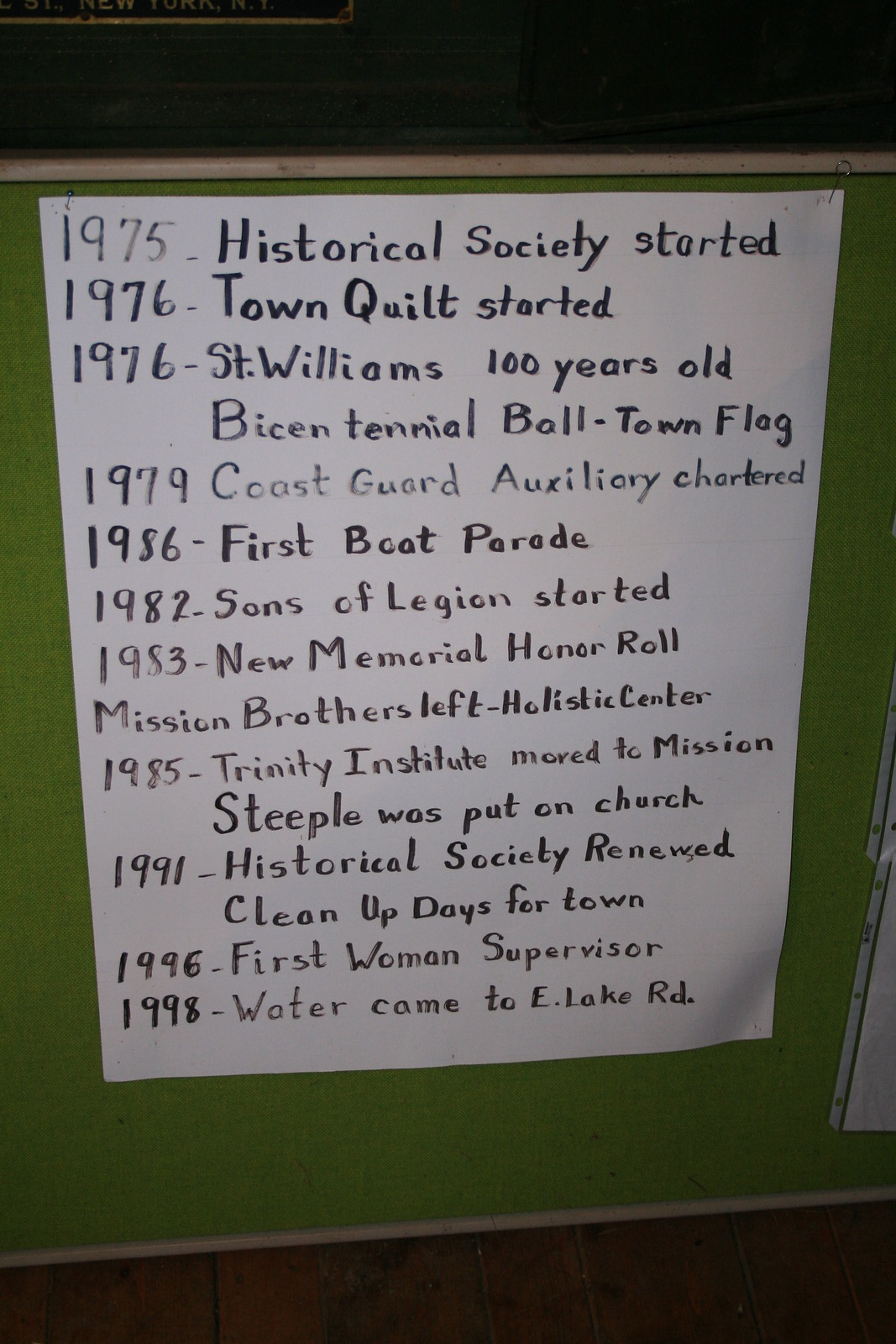The image depicts a piece of white paper tacked to a green wall with a light brown floor visible beneath. The paper contains a series of notable dates and events written in black ink. The specific entries on the paper are as follows: 

- 1975: Historical Society started.
- 1976: Town Quilt started.
- 1976: St. William's 100 years old, Bicentennial Balltown Flag.
- 1979: Coast Guard Auxiliary Chartered.
- 1982: Sons of Legion started.
- 1983: New Memorial Honor Roll, Mission Brothers left Holistic Center.
- 1985: Trinity Institute moved to Mission, Steeple put on church.
- 1986: First Boat Parade.
- 1991: Historical Society renewed, Clean Up Days for Town.
- 1996: First Woman Supervisor.
- 1998: Water came to East Lake Road.

The paper appears to serve as a historical record, listing significant community milestones over the years.